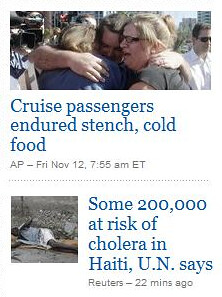The image is a close-up screenshot from a mobile news application featuring two news articles. At the top, there's a photograph depicting an emotional scene with several individuals hugging and weeping. The accompanying headline reads in clickable blue text, "Cruise Passengers Endured Stench, Cold Food," followed by the details "AP," "Friday, November 12th," and "7:55 AM Eastern" in black text. Below this, separated by a dotted black line, is another article featuring a small image of an individual lying on a hard cement ground, looking distressed. The headline, also in blue text, states, "Some 200,000 at Risk of Cholera in Haiti, UN says," with "Reuters," and "22 minutes ago" in black text underneath it. The background of the image is white and the entire layout suggests it is a screenshot from a mobile device.